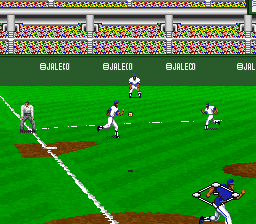This image is a vibrant, pixelated screenshot from a 1990s-era video game featuring a classic baseball scene. The scene is set on a green infield with darker green stripes diagonally oriented towards the right. The bases are marked with a reddish-brown color. Center field is alive with small, detailed figures—four baseball players and one umpire. One player, wearing a blue jersey with white pants, is running to the right. The remaining players are dressed in white uniforms with blue trim and all seem to be wearing blue caps; two are visibly running while another stands stationary. The umpire, distinguishable in dark gray pants and a light shirt, stands to the left, crouched and attentive. In the background, the stands are filled with fans, represented as colorful dots in green, red, blue, and yellow, creating a lively atmosphere. The entire scene is framed by dark green bleachers with the word "Jaleco" repeatedly printed in bold white letters across the top.